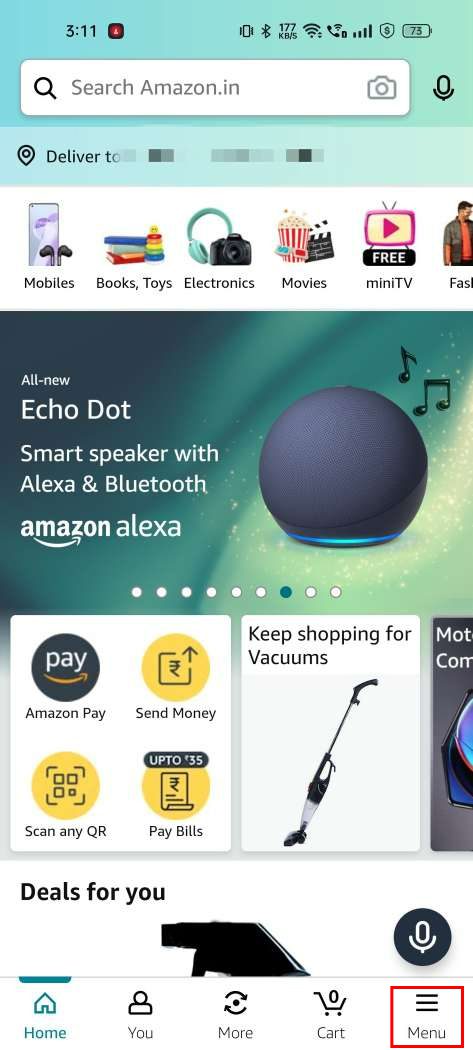Screenshot of Amazon Mobile App Interface on a Cell Phone

A detailed screenshot of the Amazon mobile app interface taken on a cell phone. At the top, the phone's status bar is visible, displaying the time on the left, followed by indicators for vibration settings, Bluetooth, Wi-Fi signal strength, and battery level on the right. Directly below, there is a prominent search bar labeled "Search Amazon.in."

Further down, the interface displays the "Deliver To" section, though the username has been blurred for privacy. Beneath this section, there are several category icons with accompanying labels and images: "Mobile" with an illustration of a phone and earbuds, "Books and Toys," "Electronics" illustrated by headphones and a camera, and "Movies" depicted with popcorn, 3D glasses, and a mini TV, alongside a "Free" label.

The next section showcases a prominent advertisement featuring the Echo Dot. It includes an image of the device and the text: "All New Echo Dot Smart Speaker with Alexa and Bluetooth."

At the bottom of the screenshot, various options are available, including "Amazon Pay," "Send Money," "Scan Any QR," and "Pay Bills," providing additional functionalities within the app.